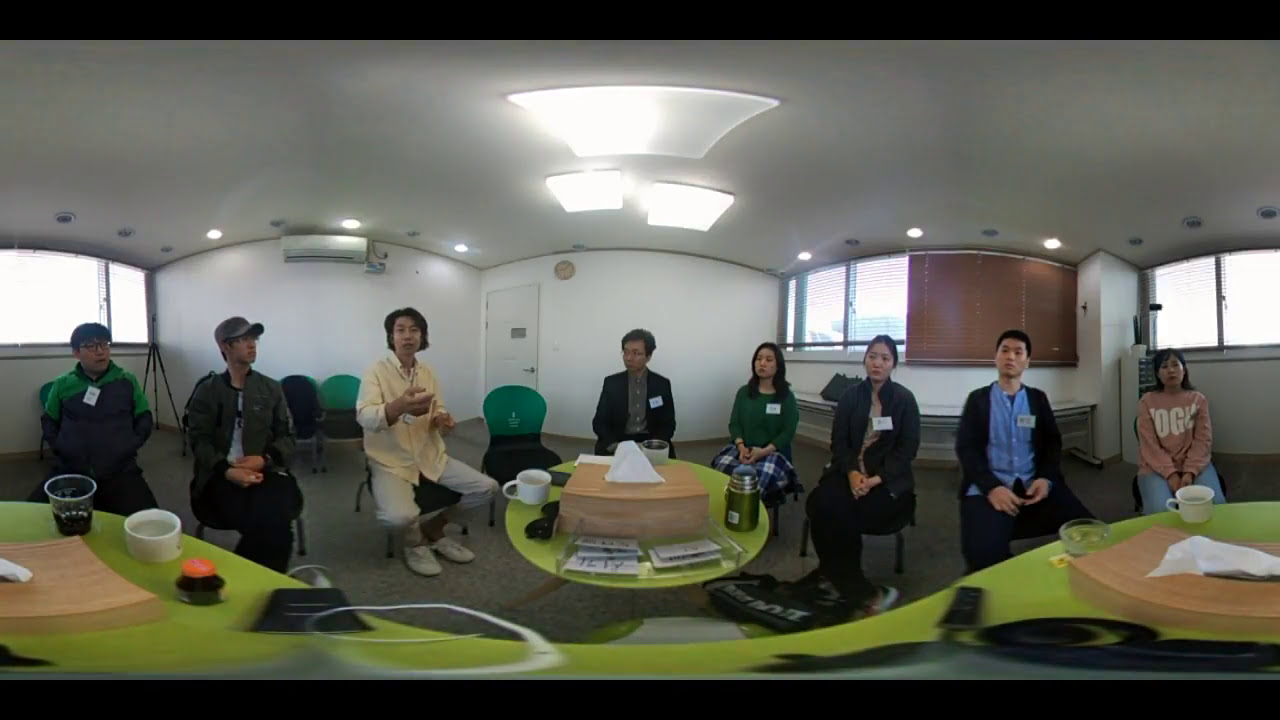The image depicts a three-dimensional panoramic view of a conference room where a business meeting is taking place. The setting is a typical meeting room with white walls, fluorescent lighting, and windows equipped with blinds on some, including wooden slats on one. At the center of the room is a round, yellow table that appears slightly distorted due to the panoramic effect. On this table, there are various items, including a box of tissues, a white mug, a teacup, and pamphlets.

Surrounding the table, seated in a circle, are eight individuals. They appear to be a mixed group of men and women, predominantly of Asian descent, and are dressed in a variety of attire ranging from business to casual. All attendees are wearing name tags on the left side of their chests, indicating their participation in the meeting. Their seating arrangement includes black chairs with green backs, and each person either has their hands folded in their laps or is holding something, possibly a drink. 

From left to right, the attendees include a woman in a peach-colored t-shirt with writing, a man in a blue shirt, a woman in a gray sweater, a woman in a green shirt, another woman in a blazer, an empty chair, a man in a yellowish shirt, a man wearing a ball cap, and a man in a blue and green jacket. One notable aspect is that the meeting environment, though professional, is quite understated with minimalistic decor and standard conference room furnishings.